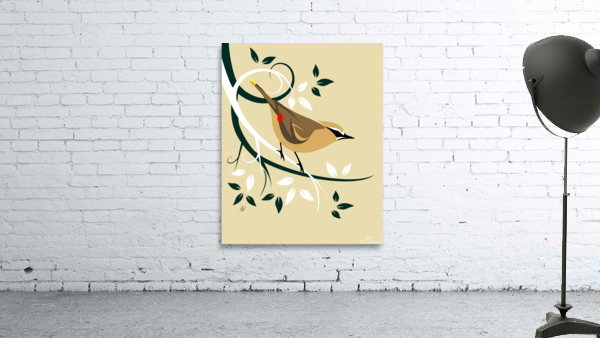The image depicts a painting mounted on a rustic, white brick wall, with some paint flaking off near the bottom, adding to an old, weathered ambiance. The ground is gray with a textured surface that could be either carpet or another material. Dominating the scene is a large painting, approximately four to five feet tall and three to four feet wide, featuring a bird perched on two contrasting tree branches—one pure white and the other pure black, creating a positive-negative silhouette effect. The bird, rendered in soft brown with darker brown wings, has distinct red tips on its wings and a yellow tip on its tail, with black eyes and beak. The background of the painting is a light, tan-like yellow, with beige and white accents. Additionally, a tall, tripod-based floor spotlight stands to the right, illuminating the painting and enhancing the details of the artwork. The overall setting is well-lit, providing clear visibility of all elements within the image.